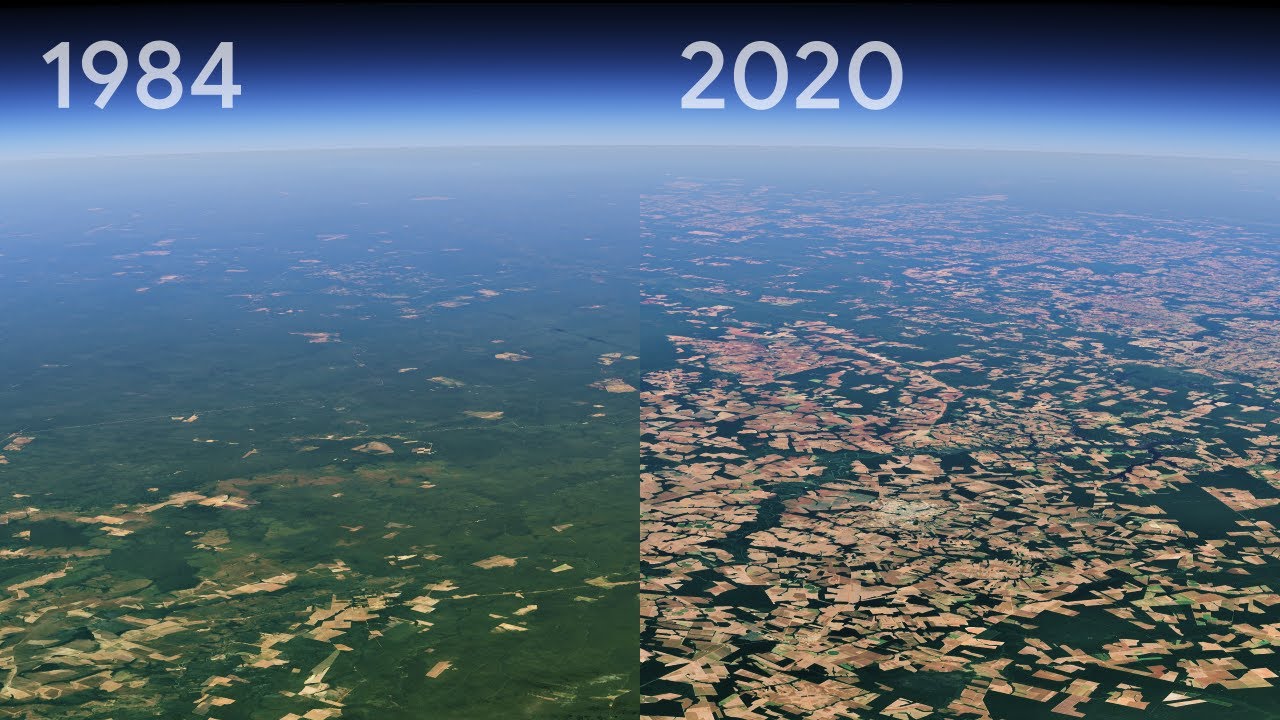The image consists of two landscape-oriented aerial photographs side-by-side, divided vertically. Both images, captured from a very high altitude, likely from a weather satellite or high-flying aircraft, offer a sweeping view of the Earth. The photographs seem to highlight the changes in a specific section of the Earth's landscape over time.

On the left, the photograph is labeled "1984" in the top left corner and displays a lush, green expanse with scattered light brown patches indicating minimal human activity or natural clearings. The curvature of the Earth is visible, blending smoothly into the blue expanse of space above, with a subtle white glow at the horizon, possibly the atmosphere.

The right photograph is labeled "2020" and depicts a dramatically altered landscape, with the green vegetation largely replaced by numerous brown and light brown rectangular shapes, suggesting extensive deforestation and land development. The brown patches are significantly more abundant and packed, indicating intensified zoning, possibly for urban or agricultural use. The curvature of the Earth and the blue of space with the atmospheric glow are consistent with the image on the left.

Together, these images starkly illustrate the impact of human activity on the Earth's surface over the span of 36 years, highlighting significant environmental changes and development.